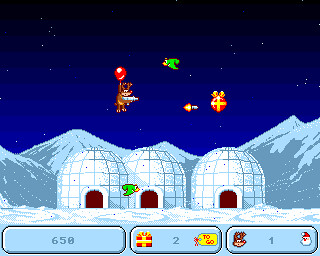The image appears to be a screenshot from an old video game, possibly designed for a handheld device. It features a reindeer character flying with the aid of a red balloon amidst a wintry landscape. The reindeer is armed with a white gun and is shooting at various Christmas presents in the sky. The backdrop comprises a gradient sky that transitions from lighter shades of blue at the bottom to darker hues, almost black, at the top. Scattered white dots depict stars in the night sky.

In the foreground, there are three igloo structures with glowing red doors, set amidst a snowy terrain. Behind the igloos, a range of snowy mountains creates a layered backdrop. Several elements are suspended in the sky, including a wrapped gift box with red and yellow stripes and a creature that could be another reindeer or perhaps a bear, all adding to the chaotic festive scene. There are green birds flying in opposite directions across the igloos, further enriching the dynamic environment.

At the bottom of the screen, score indicators and icons show game-related information. On the left, a blue box displays the number "650." The middle section features a gift-wrapped present with the number "2," and the right-side box shows a reindeer head beside Santa's head, with the number "1." The scene is bustling with activity, combining whimsical elements of Christmas and action, all set in a charming, snowy landscape.